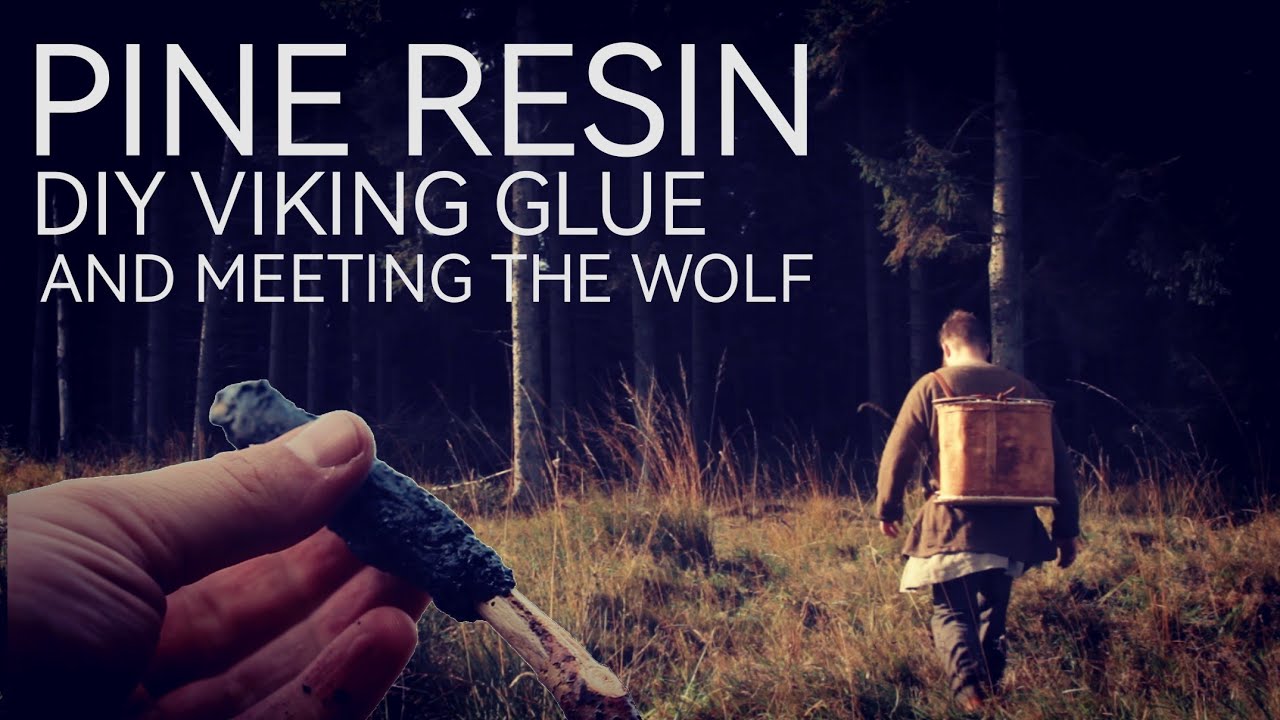This color photograph features a predominantly dark scene with a black background. Prominent white text in the upper left corner reads "Pine Resin, DIY Viking Glue, and Meeting the Wolf." In the bottom left corner, a hand extends into the frame, gripping a tool that appears to be a black-handled stick or a black screwdriver. Towards the middle right of the image, a man is seen walking away from the camera, heading towards a dimly visible forest. He is dressed in brown clothing with a white shirt peeking out under his jacket and carrying a square, primitive-looking backpack. The ground beneath him and around the scene is covered with tall, dark greenish-brown grass and weeds, which create a rugged and somewhat wild landscape.